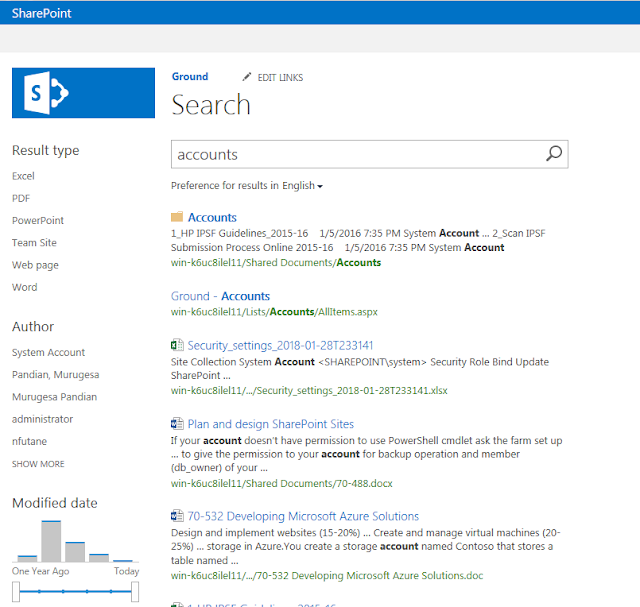This image is a detailed screenshot of a SharePoint webpage featuring a blue header. In the top left corner, the SharePoint logo is displayed prominently. The webpage is divided into two main sections. 

On the left side, there's a narrow panel with a small blue banner at the top, showcasing a logo that consists of an 'S' within a white vertical trapezoid, complete with a handle on the right side. Below the banner, the panel is organized into three sections: 
1. **Result Type** - including categories such as Excel, PDF, PowerPoint, Team, Site, Webpage, and Word.
2. **Author**
3. **Modified Date** - accompanied by a bar graph with an interactive slider at the bottom. 

The right section dominates the majority of the webpage and features a search display name above a search box. Above this search section, two texts in blue are visible, with an "Edit Links" text aligned to the right. Below the search bar, the results display five or six links. The first link is labeled "Accounts" and is sourced from "win-k6uc8ilel11," specifically mentioning guidelines from 2015 to 2016. The second link is titled "Ground Accounts" and seems to originate from a different section of the same folder. The entire webpage has a clean white background.